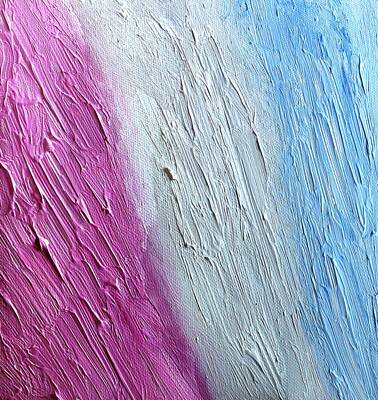The image depicts a close-up view of a textured painting, consisting of three diagonally-oriented stripes starting from the bottom left corner. The leftmost stripe is a grainy, textured pink that transitions smoothly into a central white stripe, which in turn blends into a light sky blue stripe on the right. The paint appears to be applied thickly, with brushstrokes and areas of raised paint, giving it a rough, ridged texture reminiscent of tree bark. The paint is so thick that it protrudes from the canvas or wall by about an eighth to a quarter of an inch. There is also a hint of a round metal object on the leftmost edge of the purple stripe, adding an intriguing element to the composition. The stripes are not perfectly straight or evenly divided but have an organic, geometric shape with the pink, white, and blue sections forming uneven, diagonal segments across the canvas.